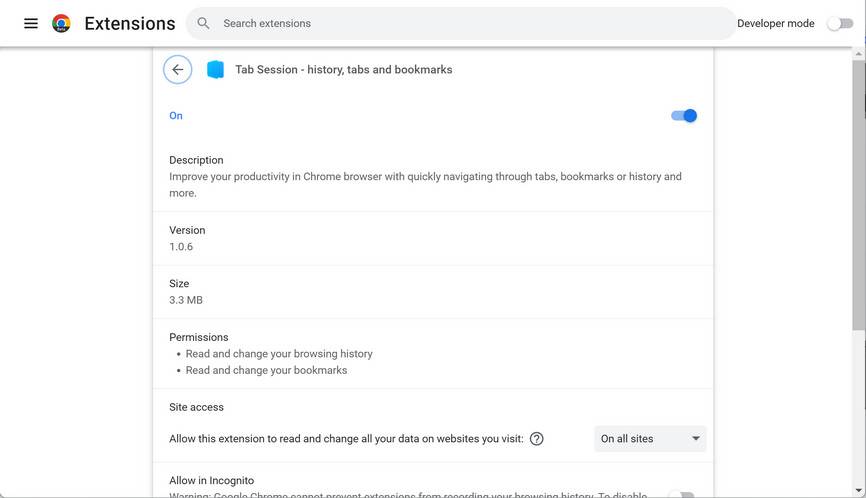The top of the interface displays the Google Chrome logo on the left, followed by the word "Extensions." To the right, there is a search bar with the placeholder text "Search extensions." Additionally, there is an option labeled "Developer mode" accompanied by a toggle switch, which is currently gray and positioned to the left. 

A gray line extends horizontally across the screen beneath these elements. Below this line, there is a circular button with a left-pointing arrow and a blue button labeled "Tab Session History, Tab, and Bookmarks."

Underneath that, in blue text, it displays the word "On," indicating that the toggle switch to the right of it is activated and blue.

Further down, there is a description stating, "Improve your productivity in Chrome browser by quickly navigating through tab bookmarks or history and more." 

Below this descriptive text, additional details are provided: "Version: 1.0.6, Size: 3.3 MB." There is also information about permissions, which include "Read and change your browsing history" and "Read and change your bookmarks." Lastly, the text notes, "Site access: Allow this extension to read and change all your data on websites you visit."